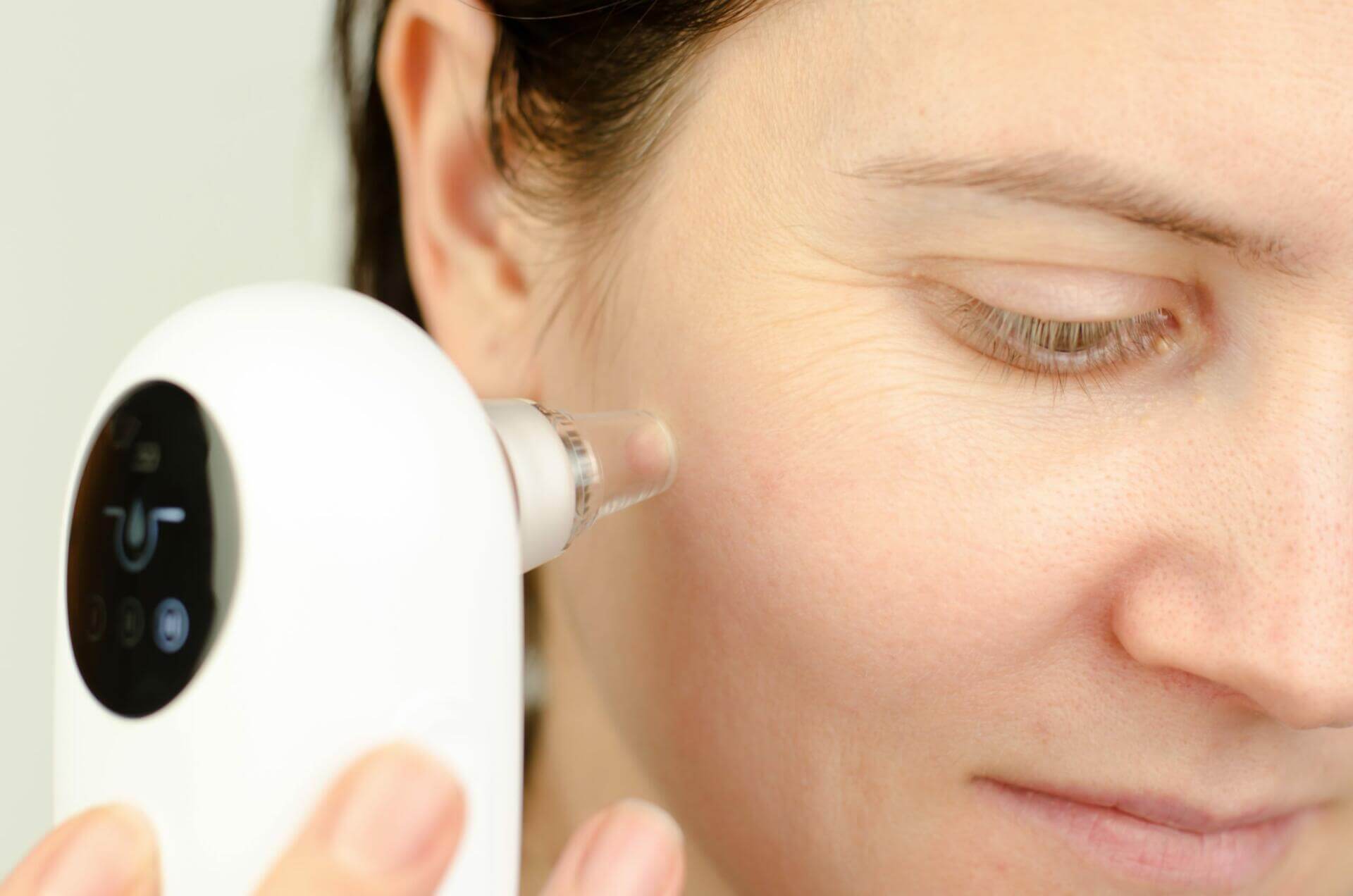In this image, a woman with short brown hair and fair complexion is captured holding a sleek, white device against her cheek. The device features a black circular screen adorned with a logo that resembles a blue teardrop and several other small symbols. The woman appears to be using this tool, which has a rounded shape and a clear tip that presses against her skin, perhaps as part of a skin treatment or to target blemishes like pimples. She is positioned near a wall, and her fingers are visible as she carefully holds the device. Although it somewhat resembles a medical thermometer, the specific usage seems to be more aligned with skincare or dermatological applications.